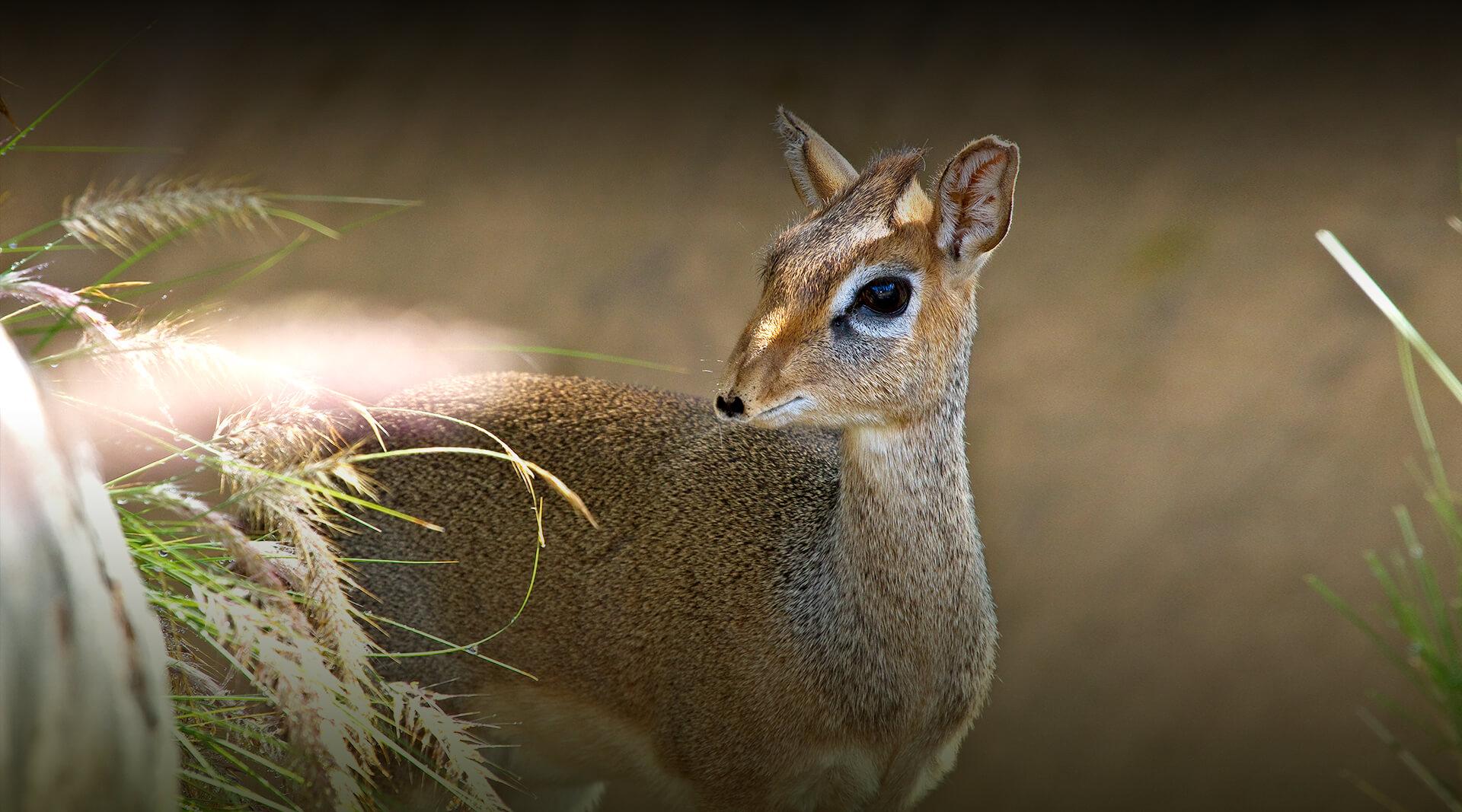The image portrays a small, young animal with characteristics resembling a deer or possibly a small antelope. The animal's fur is a mix of brown, tan, gray, and white, with distinctive white markings around its mouth and large, expressive black doe eyes that evoke a sense of curiosity and innocence. Its ears are alert, standing upright, and there is a small peak of fur on the top of its head, reminiscent of a cowlick. The animal is peeking out from behind tall grasses in a natural, sunlit setting, giving the photo a warm and peaceful ambiance. The background is blurred but features tan and green hues, suggesting a field with some wheat and grass, and there are additional elements such as the needles of an evergreen tree protruding from the right side of the image. The sunlight creates a gentle flare, contributing to the overall serene outdoor environment.